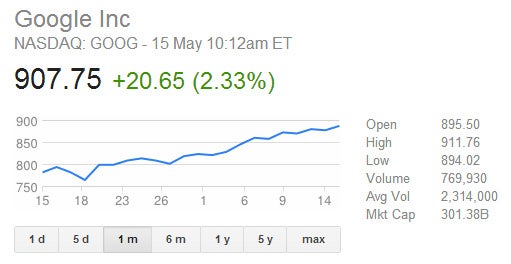This screenshot, oriented horizontally, captures the trading data for Google's stock, ticker symbol GOOG, on the NASDAQ. The upper left-hand corner of the image displays "Google Inc." and directly below it, "NASDAQ: GOOG," indicating the stock exchange and ticker symbol. The timestamp is May 15th at 10:12 a.m. Eastern Time.

The chart in the image is a simple line graph depicted with a blue line, without the specific ticker or the typical red and green candlestick pattern. The current stock price is $907.75, representing an increase of $20.65 or 2.33%, prominently displayed in green text.

On the left side of the chart, the price range is marked from $750 to $900. The x-axis at the bottom shows incremental date markings: 15, 18, 23, 26, 1, 6, 9, and 14, corresponding to days of the month. This graph represents a one-month period.

Displayed on the right-hand side are detailed statistics for the GOOG stock on this trading day:
- Opening price: $895.50
- Daily high: $911.76
- Daily low: $894.02
- Volume: 769,930 shares
- Average volume: 2,314,000 shares
- Market capitalization: $301.38 billion.